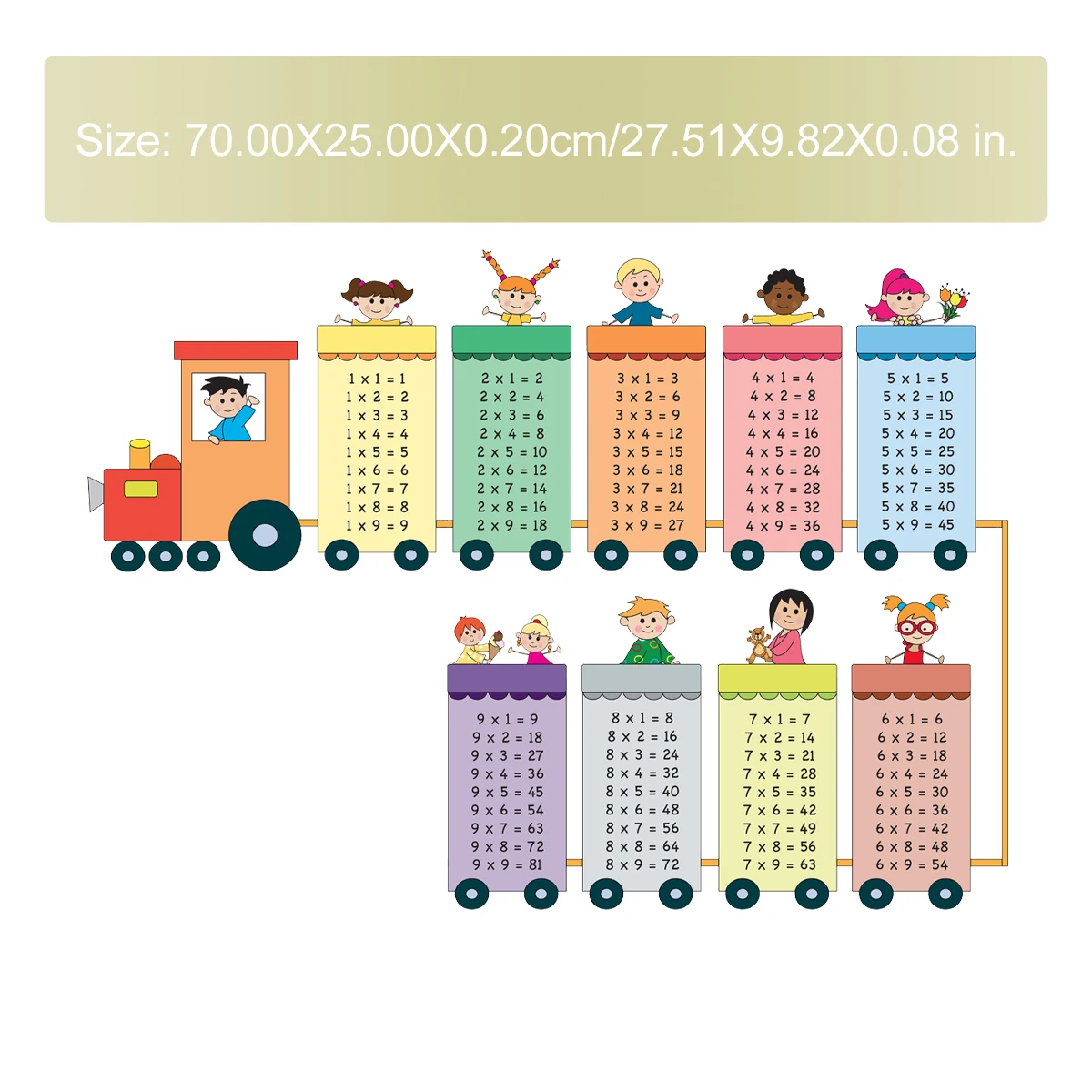The image is a classroom-friendly, cartoon-style illustration of a train designed to help children learn their times tables. The background is white, and the train, which is being pulled to the left, has a simplistic line-art style. The front cart is orange and red with large black wheels and features a young boy with a blue shirt waving. 

Each subsequent cart represents a different multiplication table from 1 to 9, with each cart in a unique color and featuring a smiling child. The first cart after the engine is yellow and displays the 1 times table up to 9, with a girl with brown hair. The second cart, featuring the 2 times table, has a girl with red hair. The third cart is orange, showing the 3 times table, with a boy with blonde hair. 

A pink cart follows with a girl who has short brown hair representing the 4 times table. After that, a blue cart has a girl with pink hair for the 5 times table. The pattern continues with each cart colorfully representing a multiplication table up to 9. 

Towards the end, a gray cart shows the 8 times table with a boy who has blonde hair. A girl with short black hair in another cart illustrates the 7 times table, and a girl with orange hair handles the 6 times table. The last cart is purple, featuring two girls with red and blonde hair, presenting the 9 times table. Each child is joyfully engaged in their respective multiplication tasks, making the image educational and visually engaging.